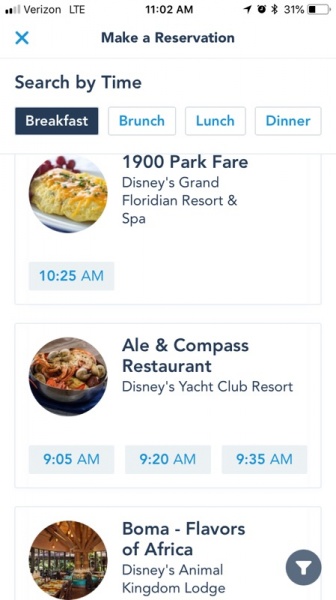In this screenshot, we see a few items related to making reservations. Starting from the upper left corner, the status bar shows three bars of Verizon LTE signal with a 31% battery level. The current time displayed is 11:02 a.m.

Below the status bar, black text reads "Make a Reservation" and "Search by Time." There are options for different meal times labeled from left to right: "Breakfast," "Brunch," "Lunch," and "Dinner," with "Breakfast" highlighted.

Just beneath this, the chosen place is "1900 Park Fare, Disney's Grand Floridian Resort & Spa," accompanied by an image of what looks like biscuits. The reservation time listed for this option is 10:25 a.m.

Following this, the next available restaurant is "Ale & Compass Restaurant at Disney's Yacht Club Resort," with available times of 9:05 a.m., 9:20 a.m., and 9:35 a.m., shown in blue text.

Lastly, the third option is "Boma – Flavors of Africa at Disney's Animal Kingdom Lodge." This section includes a round, somewhat blurry image of the interior of the restaurant.

This detailed display aims to guide users in selecting the most suitable reservation for their preferences and schedule.